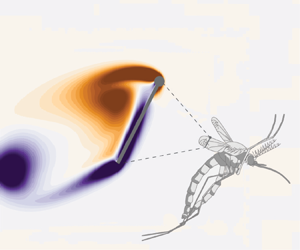The image is a square-shaped piece blending both drawing and painting techniques. Set against an ivory-toned background, the artwork prominently features a large, zoomed-in insect situated in the lower right corner. This insect, resembling a mosquito or dragonfly, is meticulously rendered in grayscale, highlighting its long thorax, two antennae, two elongated wings, and extended limbs. Just to the left of the insect is a distinctive section where traditional painting takes over. A gray line extending from one of the insect's wings forms the base of a triangle made of dotted and solid lines. 

Attached to this line is a series of vibrant, abstract shapes. A deep purple blotch extends diagonally left, tapering off into a purple blob, while shades of orange and brown intersperse around the upper and lower segments. These colorful blotches contrast against the insect's monochrome, creating a fascinating juxtaposition. The artwork's quality is high, with no text distractions, allowing the viewer to fully appreciate the intricate blend of detailed sketching and expressive painting.